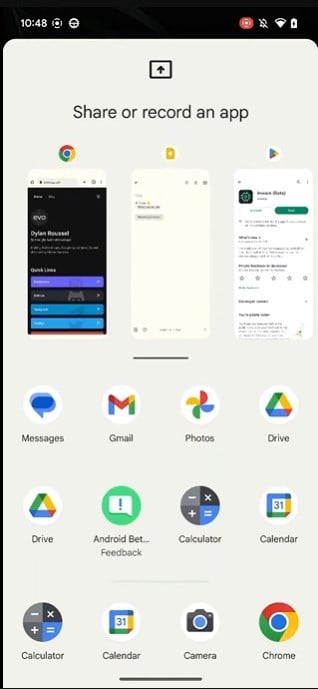The image showcases a Google smartphone with a prominent black border along the top of the screen, where the clock displays the time as 10:48 on the left, and notifications are disabled on the right. Adjacent to this, Wi-Fi strength and battery level indicators are visible. The main screen features a heading in black that reads, "Share or record an app," followed by three smaller images depicting various apps in use.

Beneath this section, there is a grid of apps, predominantly Google-related, each labeled with its respective colored icons. The first row features icons for Messages, Gmail, Photos, and Drive. The next row includes another Drive icon, something labeled Android Feedback, followed by apps like Calculator, Calendar, Camera, and Chrome. The redundancy of some apps, such as multiple appearances of Drive and Calculator, is noticeable. The consistent presence of Google logos and the variety of standard Google applications confirm that this device operates on a Google platform.